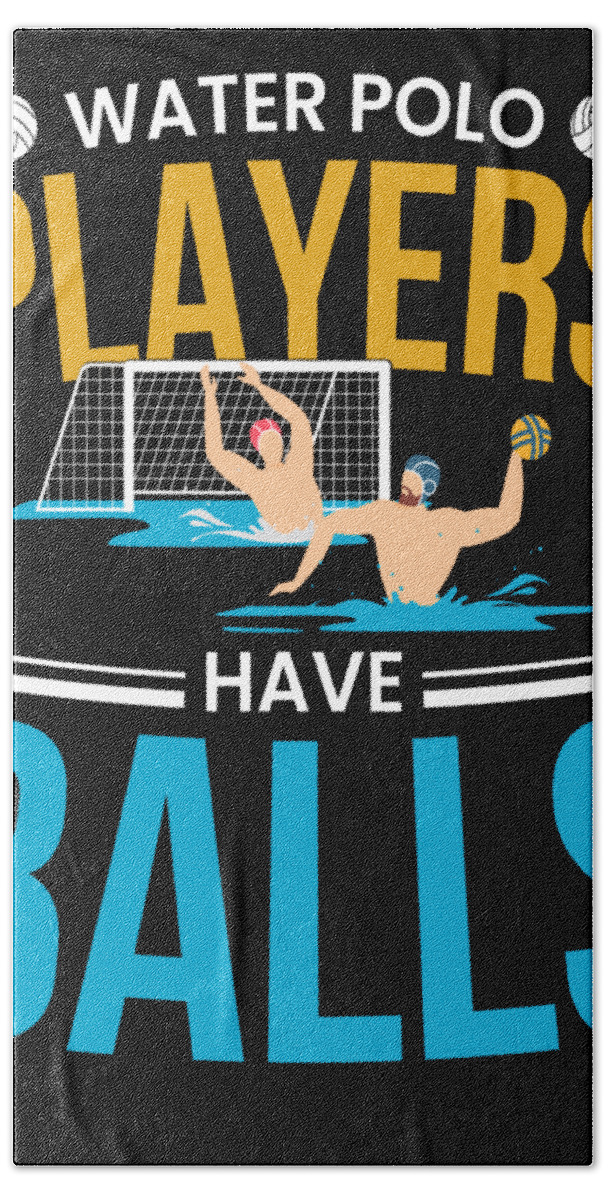The image is a vertical poster with a black, grainy background and a slightly cut-off left and right side, suggesting it might be printed on fabric or similar material. At the top, the title "WATER POLO" is displayed prominently in white, capitalized letters. Below this, the word "PLAYERS" is written in large, capitalized orange letters, but only the middle part is fully visible with the "P" and "S" partially cut off.

Central to the image are two men playing water polo in front of a white goal net. Blue water splashes around both players, indicating action. One player, with a red swim cap, is reaching up with both hands as if attempting to block or catch. The other player, with a blue cap and a brown beard and mustache, is poised to throw an orange and blue ball with his raised left hand. The scene vividly captures the intensity of the game.

Below the men, the word "HAVE" is printed in white, capitalized letters, flanked by horizontal white lines. Further down, the word "BALLS" is displayed in large, capitalized blue letters, though the "B" and "S" are slightly obscured at the edges. The overall effect is dynamic and energizing, emphasizing the spirited nature of water polo.